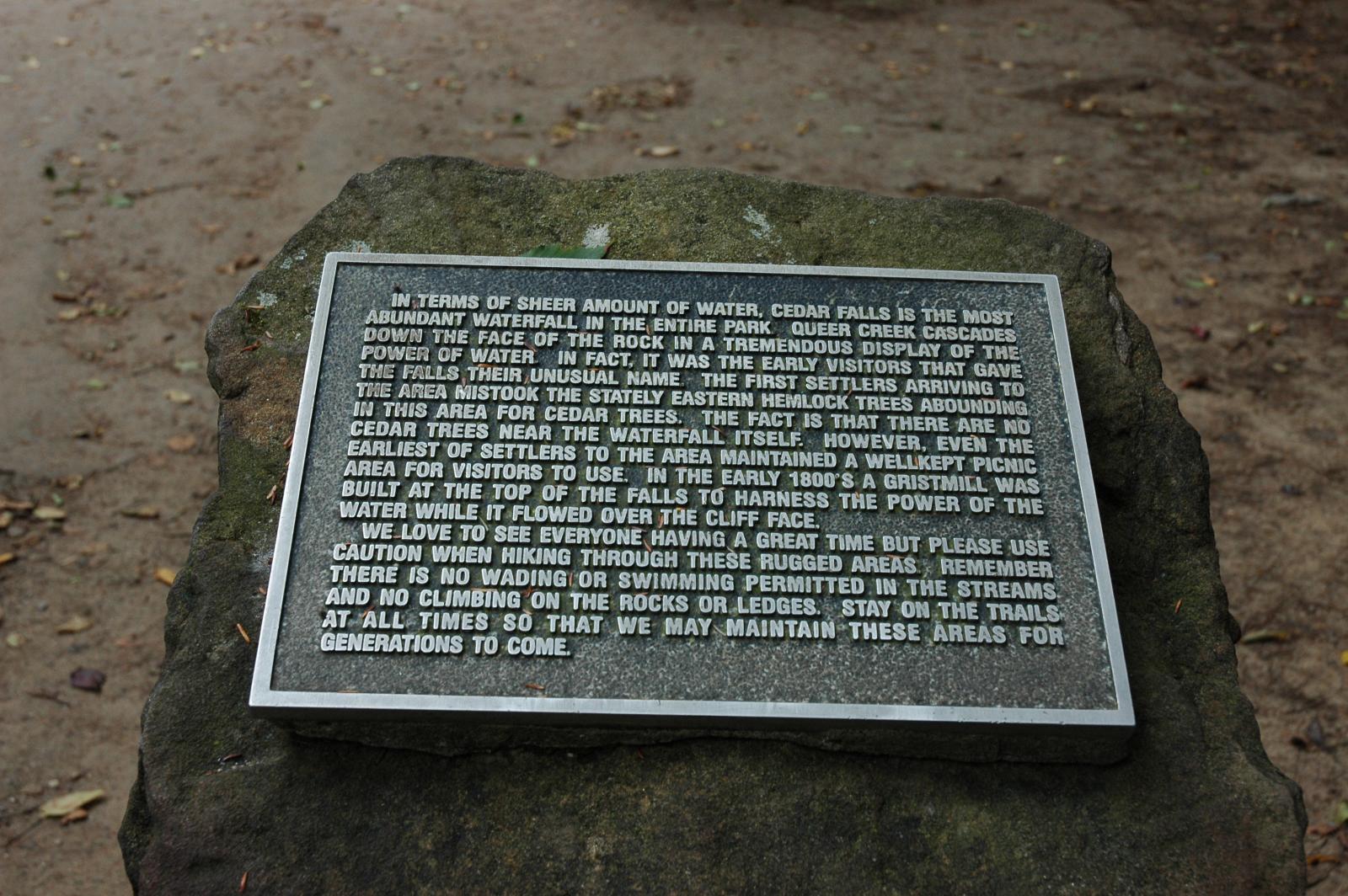This image is taken outside in a natural setting with dirt and leaves on the ground. Prominently displayed is a rock with an engraved plaque that provides a detailed historical and informational account of Cedar Falls, the most abundant waterfall in the park in terms of water volume. The plaque reads: "In terms of sheer amount of water, Cedar Falls is the most abundant waterfall in the entire park. Queer Creek cascades down the face of the rock in a tremendous display of the power of water. Early visitors to the area gave the falls their unusual name after mistaking the stately eastern hemlock trees for cedar trees. Despite this misnomer, there are no cedar trees near the waterfall itself. The earliest settlers established a well-kept picnic area for visitors, and by the early 1800s, a grist mill was built at the top of the falls to harness the water's power as it flowed over the cliff face. We encourage everyone to enjoy their time here, but please exercise caution while hiking through these rugged areas. Remember, there is no wading or swimming permitted in the streams, and no climbing on the rocks or ledges. Always stay on the trails to help preserve these areas for future generations." The setting and detailed historical context invite visitors to appreciate both the natural beauty and historical significance of Cedar Falls while ensuring its conservation.